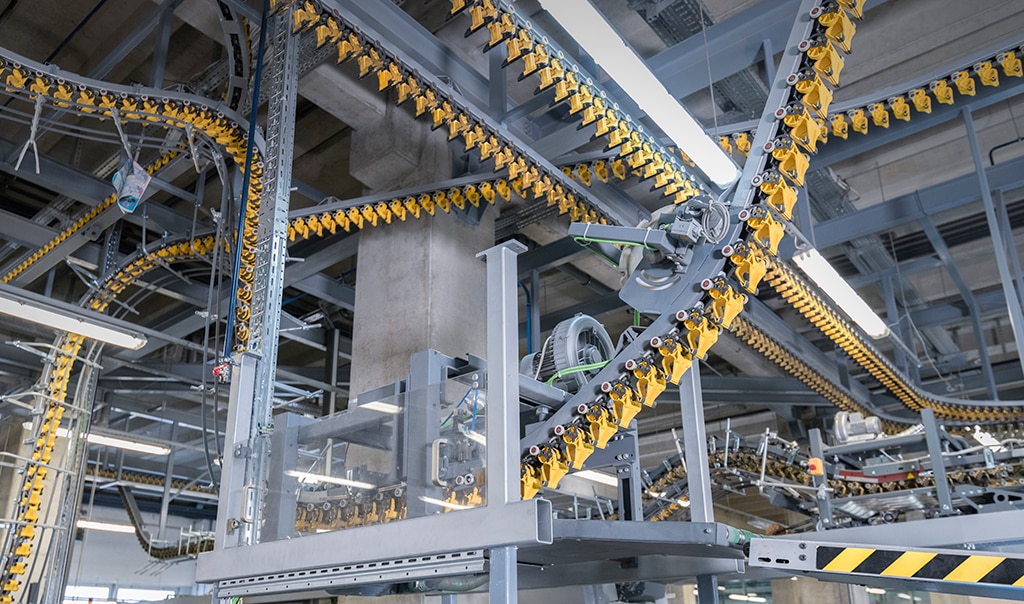The image depicts an intricate, complex assembly line within an industrial factory setting. The structure is primarily composed of gray metal beams and concrete support pillars, creating a maze-like network that spans from floor to ceiling. Numerous conveyor belts wind through the facility, resembling the tracks of a roller coaster with their straight, curved, and intersecting paths. These conveyor belts feature small yellow parts, possibly for product handling, and are integrated into the gray framework. The belts are black and yellow, and there's visible black and yellow caution tape indicating safety precautions. Additionally, a large wheel-like mechanism, potentially powering the system, is a prominent feature. The assembly line's convoluted design and the meticulous layout of machinery suggest a highly automated process within this vast warehouse or factory.